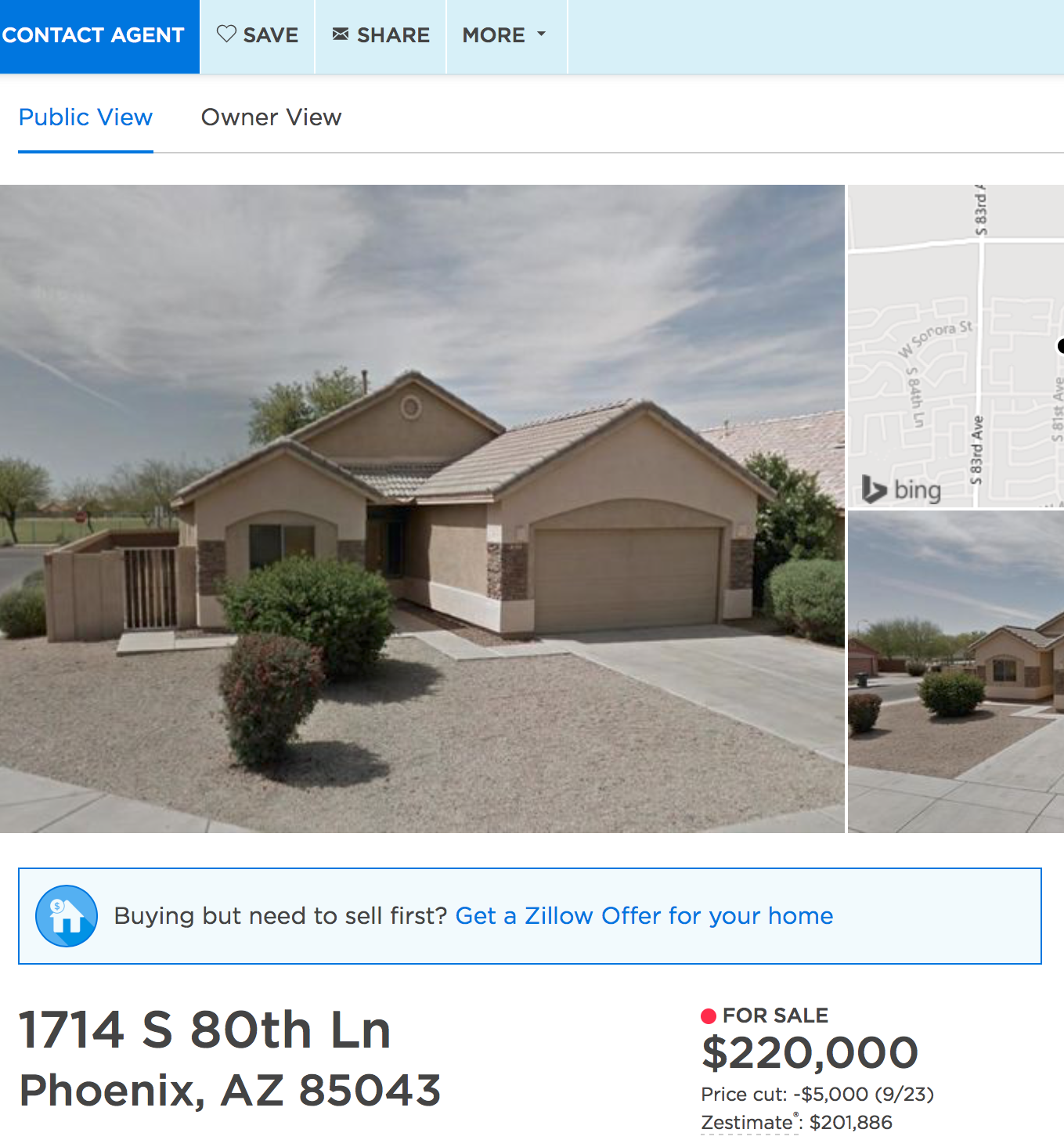This image is a detailed layout of a real estate property listing from a home selling website. The top portion of the image features a header with a light blue background transitioning into dark blue about two inches from the left. In the dark blue section, the text "CONTACT AGENT" is prominently displayed in bold, all-uppercase white letters. Adjacent to this in the light blue section, there are options listed, including "Save," an email icon for "Share," and a dropdown menu labeled "More." Below this, in a white bordered area about an inch high, there are further options including a blue underlined "Public View," and next to it, "Owner View" written in black.

The main body of the image displays a picture of the house, which spans approximately three-quarters of the way across from the left side. The house is brown with a darker brown roof and garage. The front yard is composed of gravel with a long driveway and a cloudy sky as the backdrop. Two bushes are visible in front of the house on the left side. To the right of the house image, there is a map situated in the bottom left corner with the label "Bing" below it. 

Below this area is another picture of the house followed by a large blue rectangle that spans the width of the image. This rectangle has a dark blue border and a light blue interior. On the left side of the rectangle, there is a blue circle featuring a white house icon. To the right of this icon, the text reads: "Buying but need to sell first?" in black, followed by "Get a Zillow offer for your home" in blue.

In the section beneath this, on the left side, bold black lettering shows the address "1714 S 80th LN" with "Phoenix, AZ 85043" displayed right below it in slightly smaller but still bolded black text. On the right side of this information, there is a red dot followed by the words "For Sale" in small letters. Below this information, in larger font, is the price "$220,000," followed by "Price cut $5,000" underneath it. Lastly, the estimated value "$201,886" is also shown.